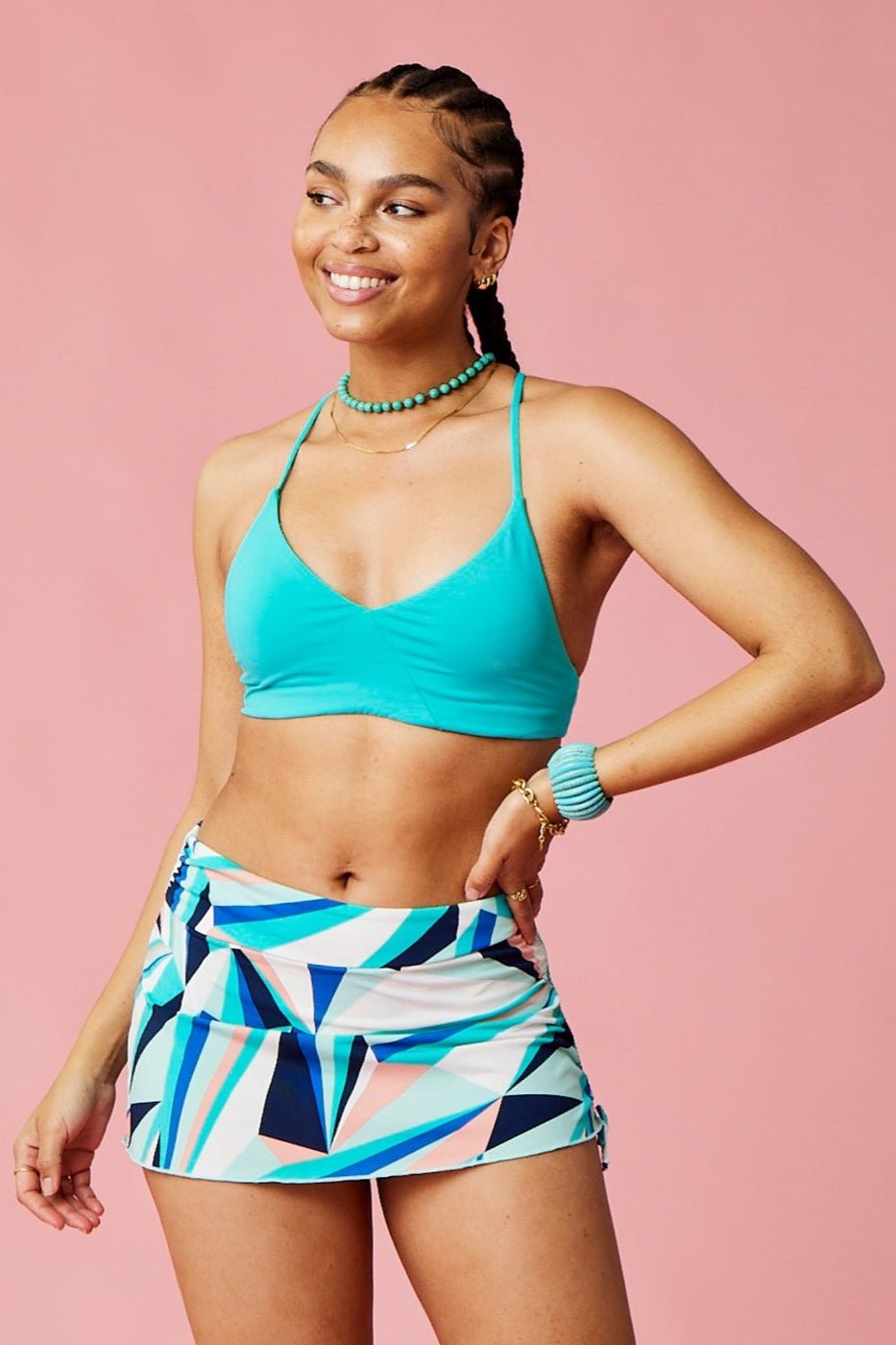This professional color photograph captures a young, slender African-American woman, likely in her late teens to mid-twenties. She stands confidently against a solid pink background with a warm, radiant smile directed slightly to the left. Her neatly braided hair is pulled back, accentuating her delicate features and light brown complexion. She is adorned in an aqua-colored ensemble that includes a crop top or sports bra, a beaded necklace, and a matching bracelet, which create a cohesive look. Her mini skirt is decorated with a vibrant array of geometrical shapes in hues of blue, green, pink, peach, and white, adding a dynamic flair to her outfit. Her hand, adorned with rings and an additional gold bracelet, rests confidently on her hip, highlighting her toned physique. The lack of text suggests the image may be used for a clothing advertisement, although this remains open to interpretation due to the absence of specific context.